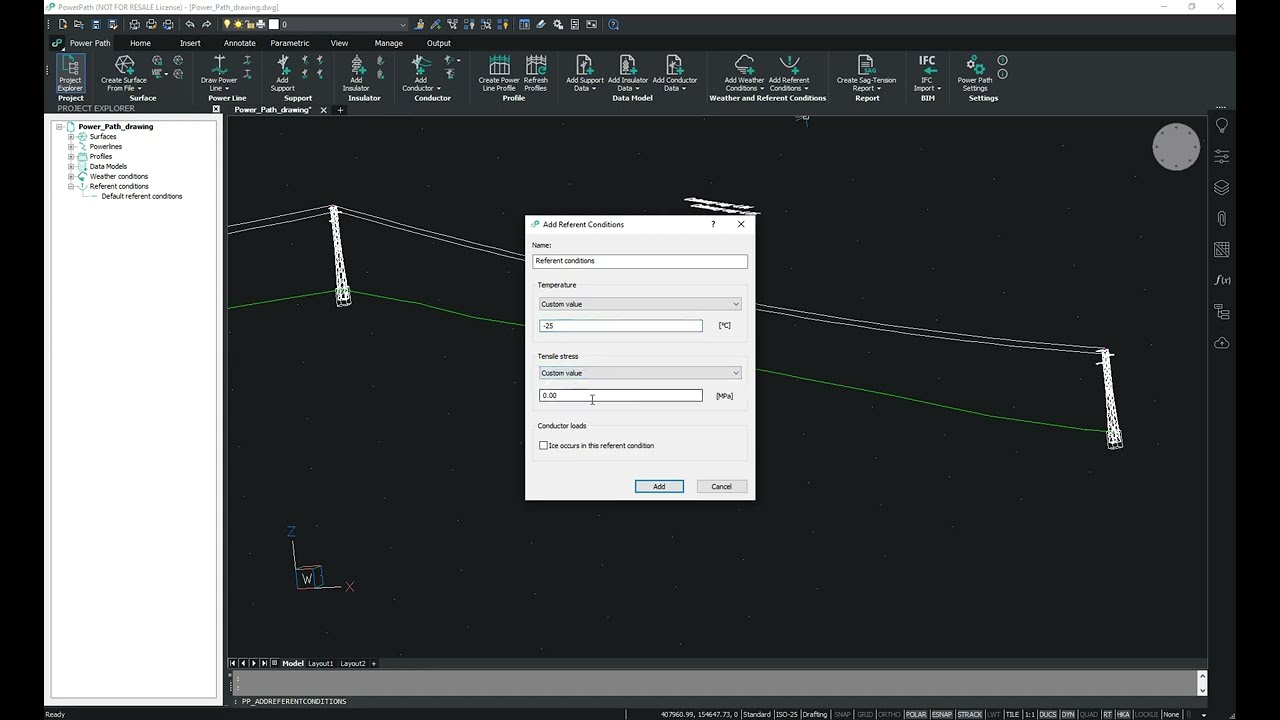This image is a detailed screenshot from a computer showing a graphic design application, likely related to engineering or technical drawing, possibly using a software named Power Path. Dominated by a theme of black, white, and gray, the screen also features accents of blue, yellow, red, and green. At the top, there's a comprehensive toolbar with numerous tiny symbols and text, though the specifics are unreadable due to size. Centrally, there is a prominent gray dialog box labeled "Referent Condition," which includes various customizable fields such as "Temperature Custom Value" (with a unit in Celsius), "Stress," "Conductor Load," and "Ice Occurs." On the left, there is a white menu list with options like "Power Path Drawing," "Surfaces," "Power Lines," "Profiles," "Data Modes," and "Weather Conditions." Although the visual information is abundant with multiple lines and shapes hinting at some form of graph creation, the overall precise functionality remains partially obscured by the lack of legibly detailed text.